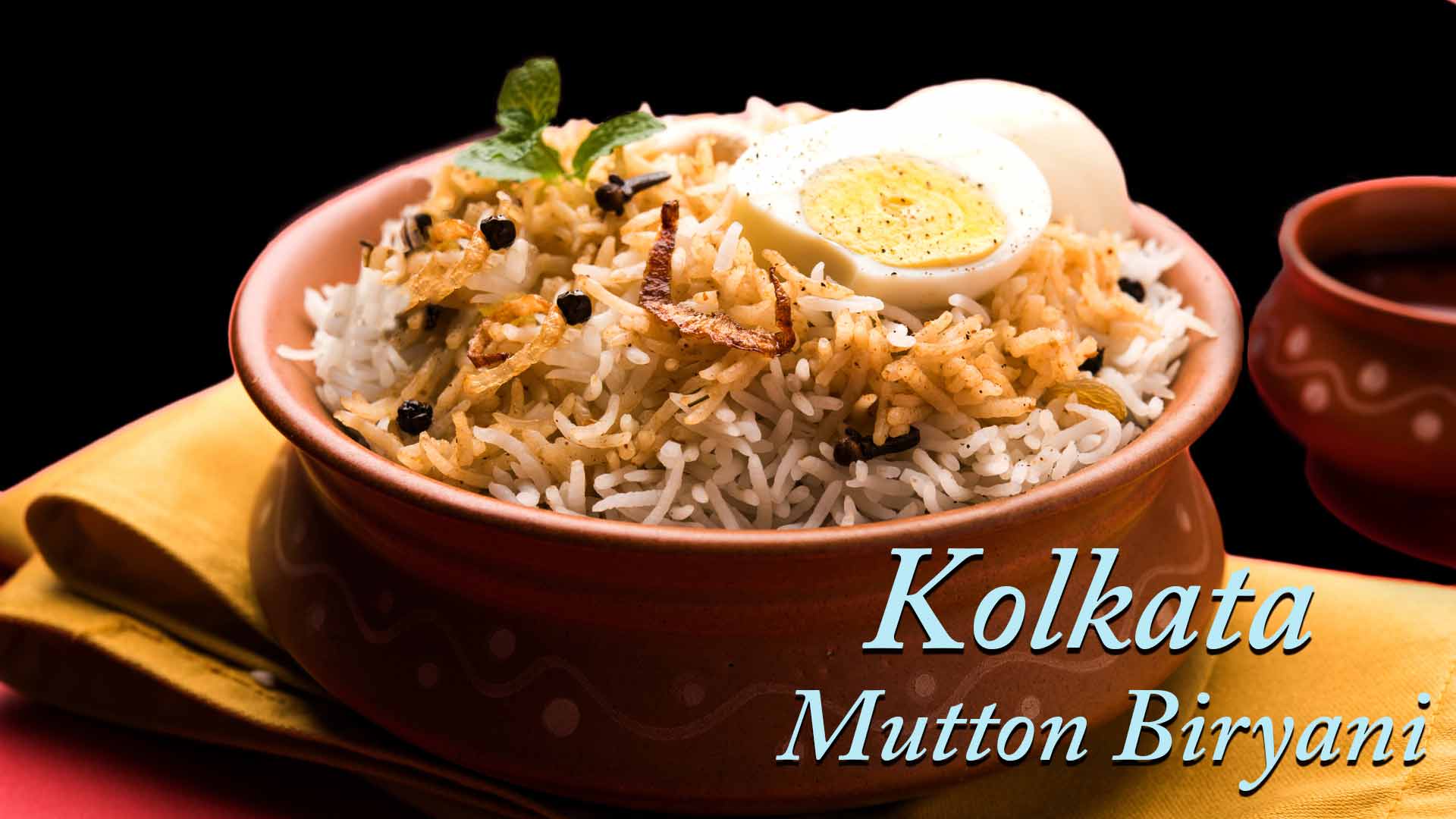This professionally staged, full-color photograph showcases a bowl of Kolkata Mutton Biryani, prominently labeled in light blue text in the lower right corner. The dish, presented in a brownish-orange, porcelain bowl, features both white and brown rice, sprinkled with seasoning. Atop the rice sits a hard-boiled egg, meticulously sliced in half to reveal its hardened yolk, and garnished with what appears to be basil. The bowl rests on a neatly folded yellow dish towel atop a red surface, likely a table. In the far right, another bowl of a similar color and design is visible but empty. The image is set against a completely black background, which enhances the vivid colors and detailed textures of the food and table setting.